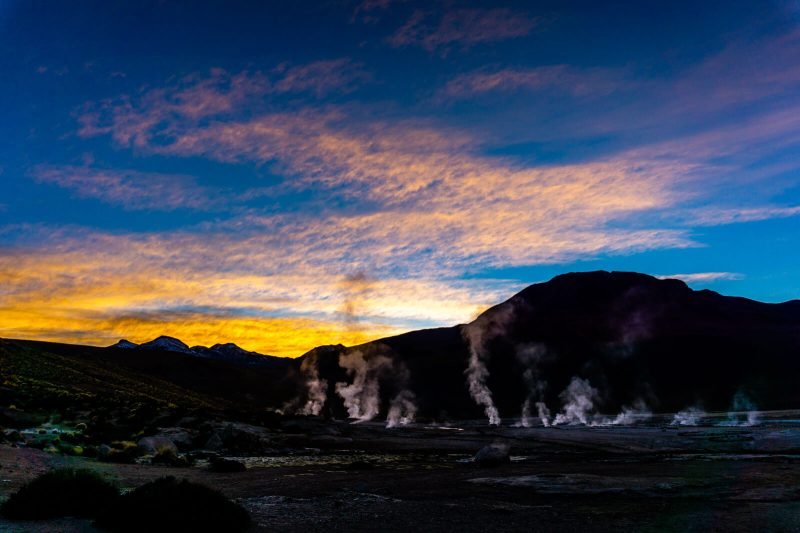This photograph captures a blurred yet enchanting sunset landscape. The sky transitions from a bright blue at the top to a hazy white with wispy clouds, tinged with orangey-yellow hues near the horizon, reflecting the setting Sun. The background features dark rolling hills and a prominent rocky formation silhouetted against the colorful horizon on the left. The foreground is dominated by a dark, shaded area that seems to be a flat plateau, with a mixture of brown or gray dirt, some gray rocks, and sparse shrubs. Notably, thin wisps of smoke or steam rise mysteriously from the ground, reminiscent of geysers or hot springs, adding an ethereal quality to the scene. The overall image conveys a sense of twilight, with its dark, silhouetted elements contrasting beautifully with the vibrant evening sky.